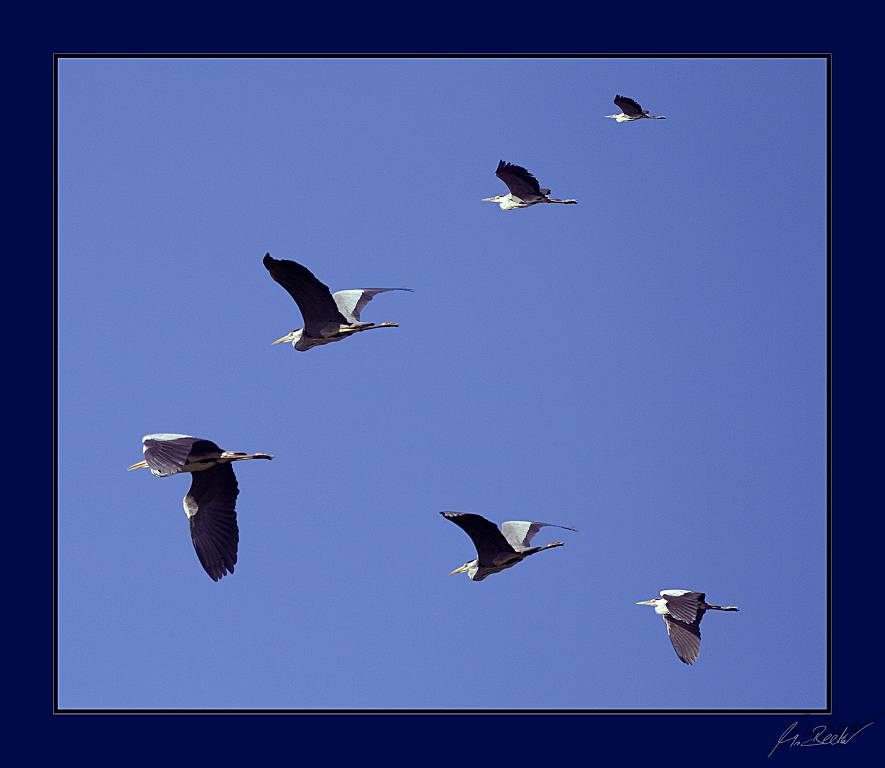The image is a square color photograph, elegantly framed with a dark blue border, and signed at the bottom, possibly with the initials "J.R.B." or "J.BECH." The focus of the photograph is an array of six birds in formation, flying from right to left against a perfectly clear, blue sky. The birds, which appear to be geese, are forming a V-shaped pattern with the lead bird positioned at the bottom right. They have distinct black undersides to their wings and stark white tops, along with white heads, beaks, and chests. Sunlight illuminates their wings, creating a striking contrast between the black underside and the bright white tops. This detailed scene captures a moment of coordinated flight under the brilliance of a sunny, cloudless day.